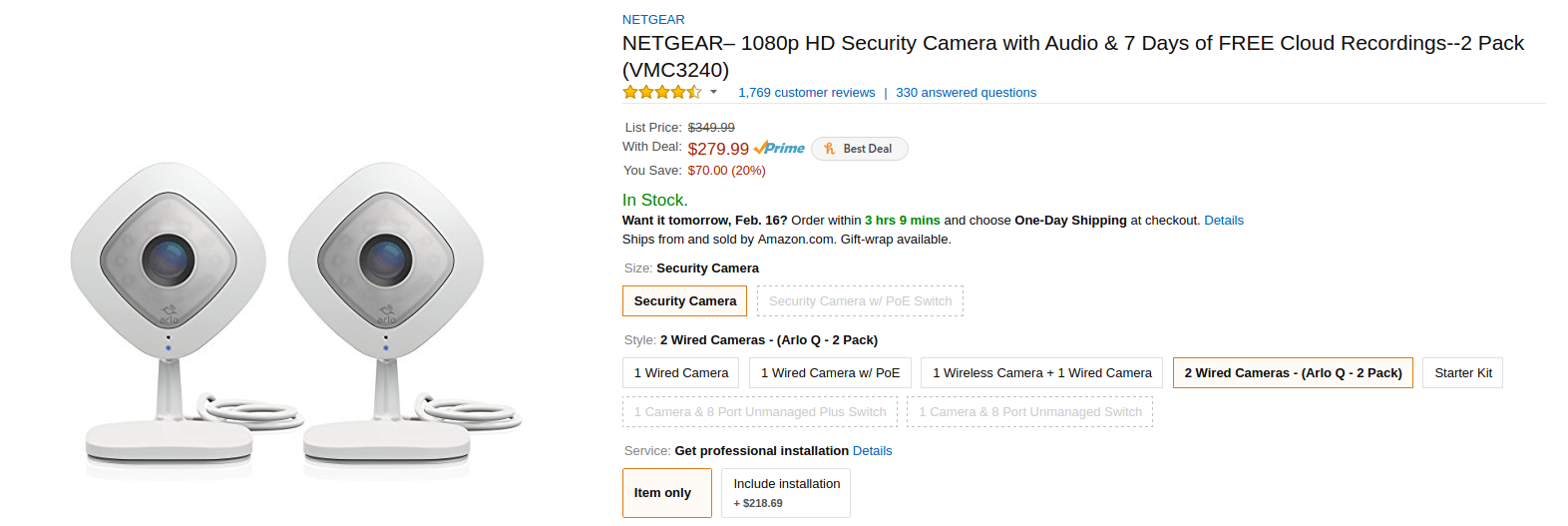This image is a screenshot of an Amazon listing for a Netgear security camera system. The product is advertised as a "Netgear 1080p HD Security Camera with Audio and Seven Days of Free Cloud Recordings." It comes as a two-pack, providing two cameras for enhanced security coverage. The listed price is $279.99, and the product is currently in stock, highlighted in green letters.

The listing emphasizes that the item is available with Prime shipping. A specific prompt in green informs customers that if they want the product by tomorrow, February 16, they need to order within three hours and nine minutes and opt for one-day shipping at checkout. Notably, the word "Details" is in blue, indicating an interactive link for more information.

The description clarifies that these are two wired cameras offered in the two-pack. For those requiring assistance, professional installation services are available for an additional $218.69. The listing's background is white, with the primary text in black. Colors such as blue for links and green for stock and shipping information provide visual cues for navigation and product availability.